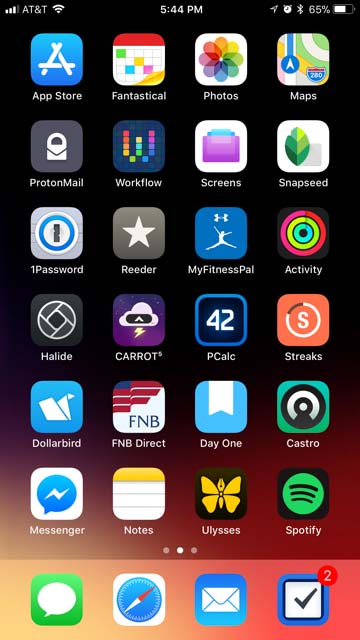The image is a detailed view of a smartphone screen, either an iPhone or an Android device, depicted in a vertical format. The background starts with a dark, black hue at the top, gradually transitioning to a reddish color toward the bottom right corner.

At the very top of the screen:
- The left corner displays a white icon indicating three out of four cellular signal bars.
- Adjacent is the 'AT&T' carrier name in white.
- Further right is a white Wi-Fi symbol.
- Centered at the top is the time, "5:44 PM", in white.
- To the right, there is an array of icons: an upward-facing triangle, an alarm clock symbol, an unidentified gray and white icon, followed by a battery icon showing "65%" with a partially filled battery.

Below the status bar:
- There are six rows, each containing four app icons with their names underneath in white text.
- Notable apps include the Google Photos icon (third from the left in the top row) with its multicolored pinwheel on a white background labeled "Photos."
- In the penultimate row, there’s the Messenger app, represented by a white square with a blue speech bubble containing a white lightning bolt, next to the Notes app.
- The upper rightmost icon is identified as the Google Maps app.

At the bottom:
- Three dots are visible, where the two dots on the sides are pink and the one in the middle is white.
- Below the dots is a long pink navigation bar, darkening toward the right.
- From left to right, the navigation bar includes four icons: 
  - A green square with a white speech bubble.
  - A white square featuring a blue compass with a red needle.
  - A blue square containing an envelope icon.
  - A blue outline square with an internal black-rimmed square, white interior, black checkmark, and a red circle with the number "2" in the upper right corner.

The screen provides a snapshot of various popularly recognized and unrecognized app icons, exemplifying a diverse collection of applications installed on the device.